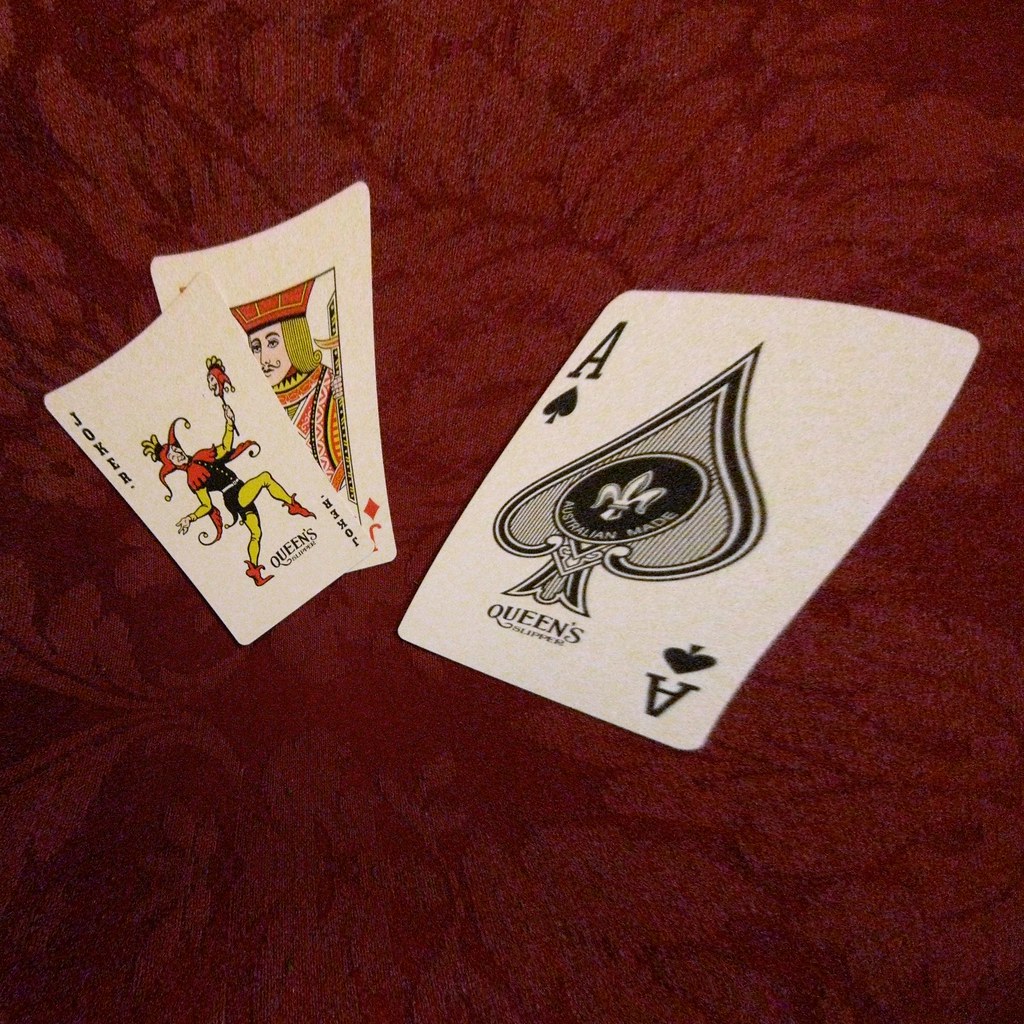This is an image of three intricately detailed playing cards, displayed on a rich red background, possibly a blanket. The cards appear slightly warped, either due to the camera lens or their own wear, with a wavy, somewhat distorted appearance. The prominent card in the forefront is an Ace of Spades, notable for its large size and elegance. It features "QUEENS" inscribed beneath a black spade which contains a fleur-de-lis symbol at its center, contrasted against a white background.

Behind the Ace of Spades, there are two overlapping cards. The upper card is a Joker, adorned in a vibrant red, yellow, and black outfit. The word "QUEENS" is also present beneath the image of the Joker, adding a unique touch. 

The third card, partially obscured by the Joker, is a Jack of Diamonds. Positioned diagonally, only the upper half and the bottom-right corner are visible, clearly indicating its suit and rank. The image captures a sense of curiosity and mystique, enhanced by the slightly bent and irregular shapes of the cards.